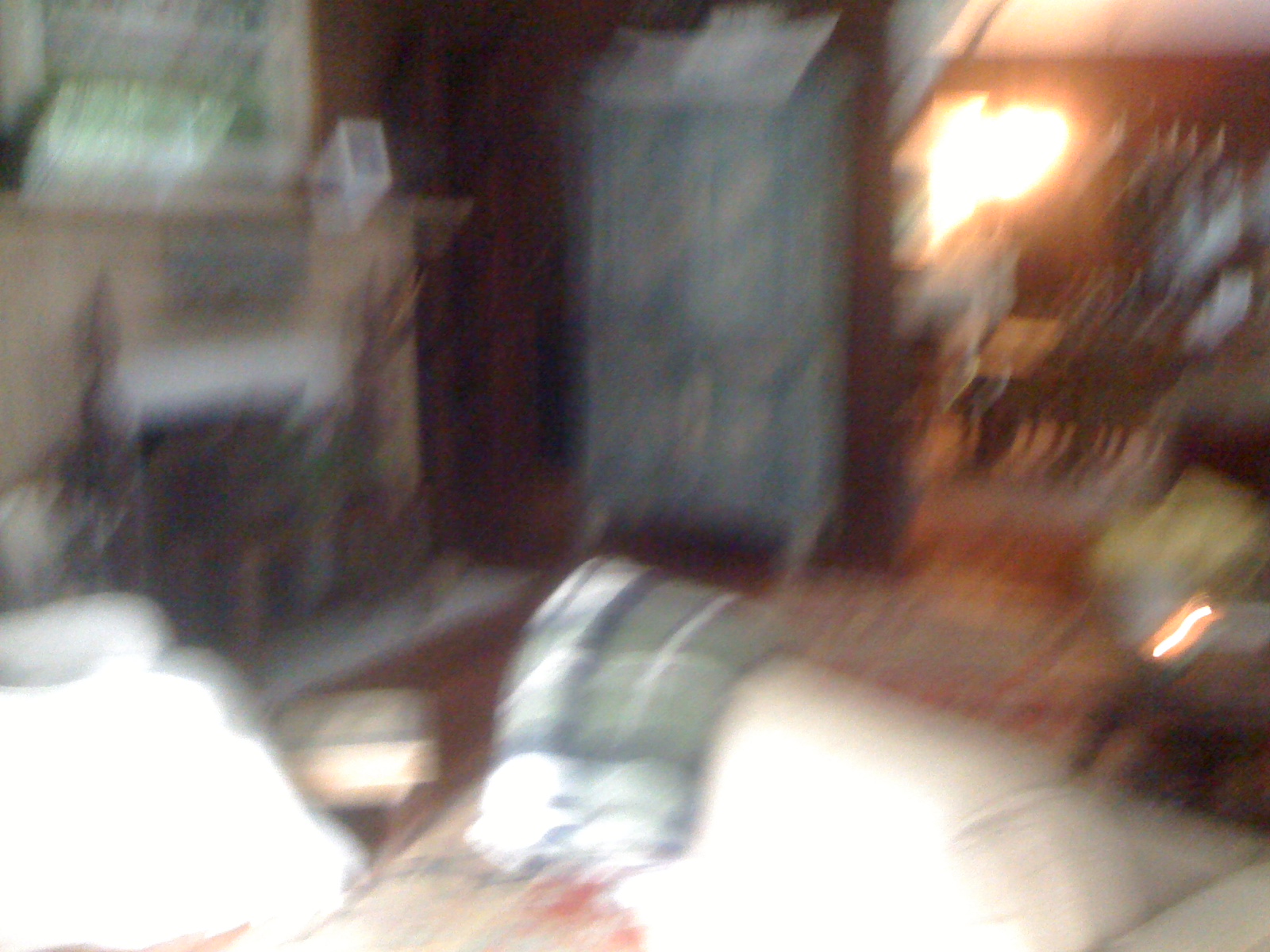A blurry image appears to capture a section of a house, likely the living room. On the left side, there's a fireplace adorned with a white picture frame on the mantle and flanked by green items or perhaps a large picture frame that reflects something indistinct. The fireplace is surrounded by white trim and is accented by brown details. To the right, a substantial blue piece of furniture, possibly a closet, stands against a brown wall. Beyond this, a dining area is visible with a brown dining table and illuminated by a yellow light against a red wall. The ceiling above the dining area is white. In the foreground, there's a pillow or folded sheet in shades of green, blue, and white. The bottom left corner of the image is dominated by an indiscernibly bright white object. The entire photograph is notably blurry, making finer details difficult to discern.